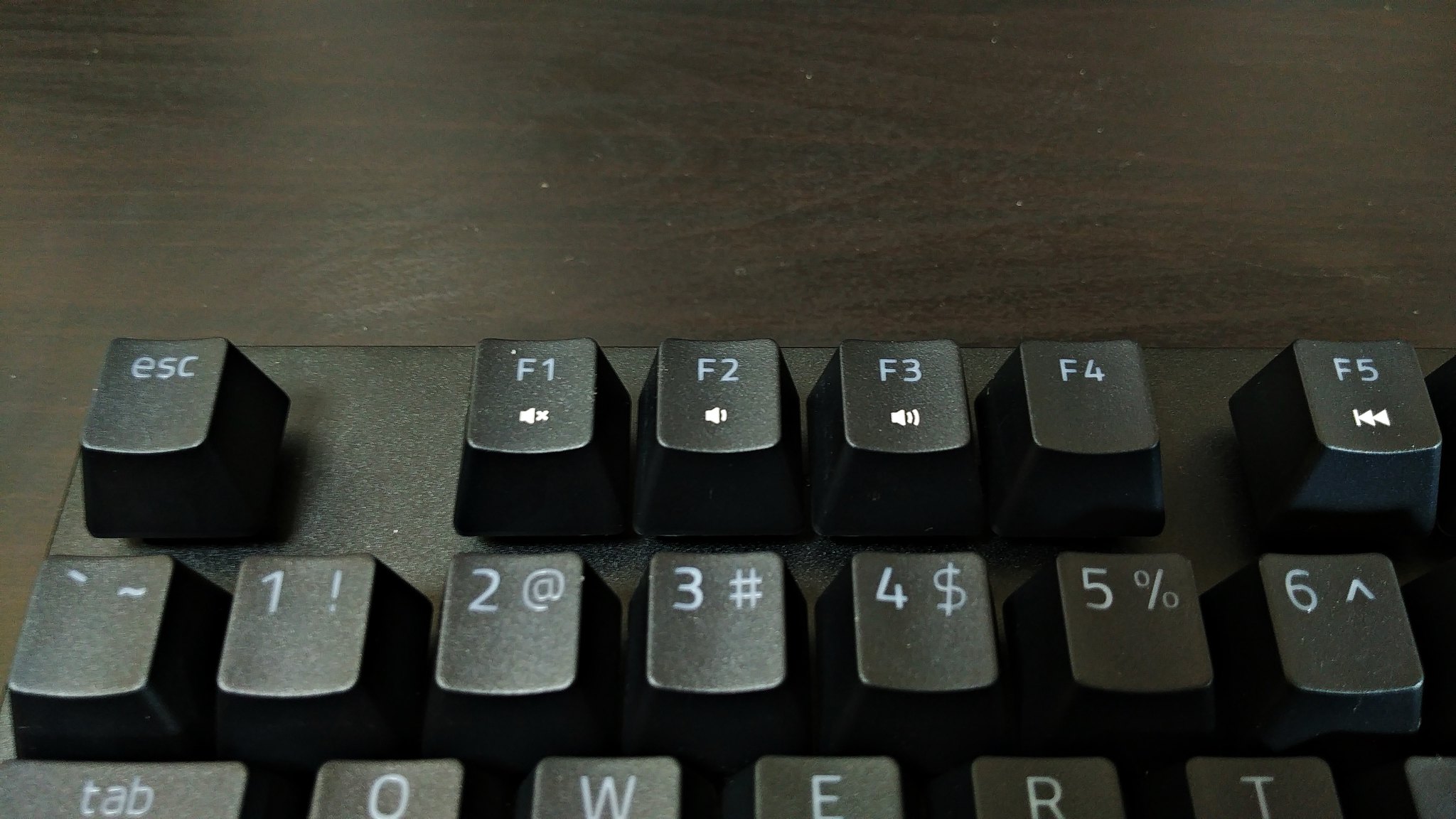This horizontal rectangular color photograph presents a realistic close-up of a black plastic computer keyboard set on a dark, almost black wooden surface, likely a desk or table. The photograph features the upper left-hand corner of the keyboard, revealing three partial rows of raised keys. The keys, which are black with white labels, include the ESC key, F1 through F5, the tilde, the numbers 1 through 6, and the letters Q, W, E, R, and T. The image is shot in landscape mode, making it wider than it is tall. There are no additional markings, people, or animals in the photograph.